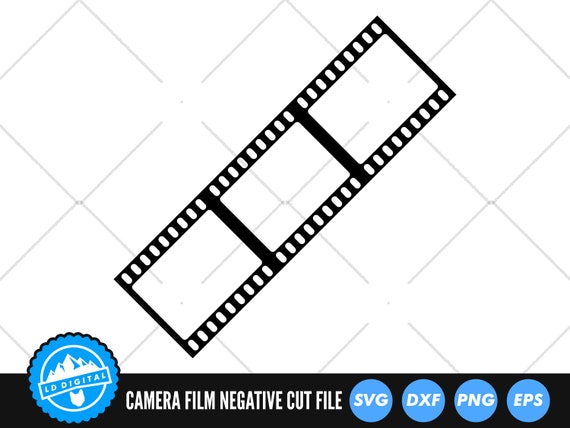The image features a white background with diagonal gray squares running across it. Centrally positioned is a piece of black film strip, reminiscent of old movie reel film, extending from the bottom left to the upper right. The film strip frame is empty with little black dots on the sides, enhancing its appearance as a classic film negative.

At the bottom of the image is a long black rectangle. On the left side, there's a blue circular logo with a white mountain and a white surrounding circle, labeled "LD Digital." To the right of the logo, in white capital letters, it reads: "CAMERA FILM NEGATIVE CUT FILE."

Further to the right of the text are four blue circles, each containing white letters from left to right: SVG, DXF, PNG, and EPS, indicating the file formats available. The overall image skillfully combines white, black, and blue elements, creating a striking, vintage-inspired graphic.